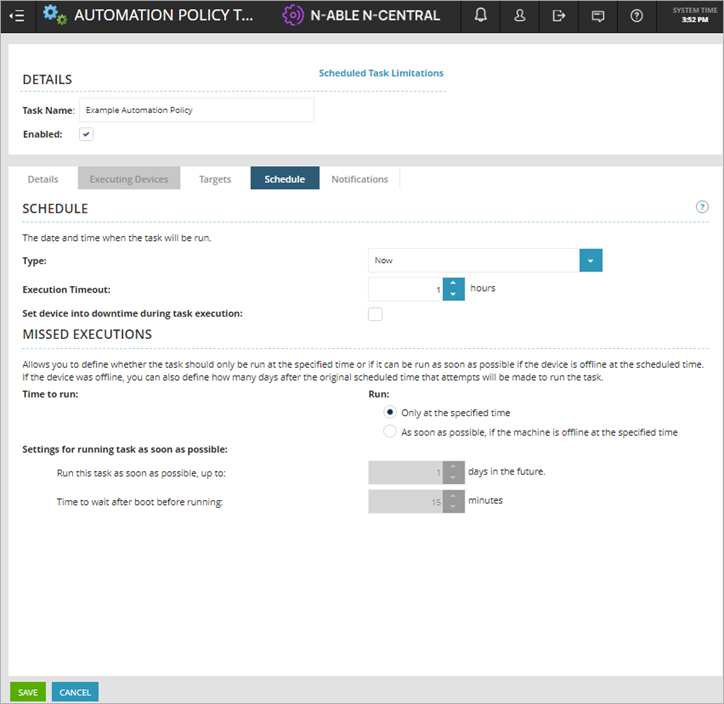A detailed screenshot of an automation policy website interface. 

The background predominantly features a clean, white layout. At the top, there is a black horizontal menu bar with white text. On the far left, three horizontal bars indicate a menu for additional options. Adjacent to this, the company's icon—a pair of interlocking gears with the larger one in blue and the smaller one in green—is displayed. Beside the icon, the text "Automation Policy T..." trails off in white. 

Close to this text, a purple icon contains a gear on the left side and extends into curved sound wave lines on the right. Adjacent to this, it reads "N-ABLE N-CENTRAL" in white. Moving to the right side of the menu bar, there are several icons likely representing notifications, user count, sign out, messaging, and help options. 

Further to the right, the system time is displayed in medium gray, reading "3:52 p.m." underneath. 

The central section of the screen contains multiple tabs labeled "Details," "Executing Devices," "Targets," "Schedule," and "Notifications," indicating various categories of information about scheduling and execution details. This area is cluttered with black text, dropdown menus, and text fields providing comprehensive options and settings.